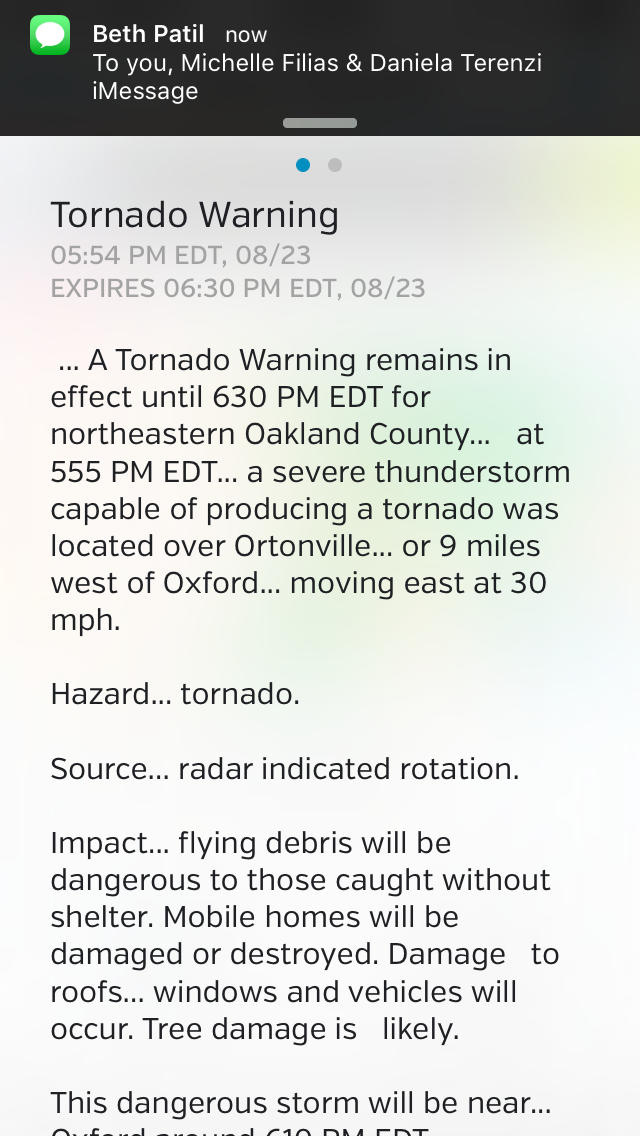This vertical rectangular image depicts a screenshot of a text message on a cell phone. At the top, there is a small black bar, roughly one-sixteenth of the image, containing the green and white messaging app logo on the left. Next to the logo, text in white reads, "Beth Patel to You," followed by "Beth Patel now to You, Michelle, Phyllis, and Danielle Tervenze," indicating the sender and recipients.

The body of the message, displayed below in white text on a gray background, begins with a time stamp: "5:54 PM EDT, 08/23," and an expiration time: "6:30 PM EDT, 08/23." The text reads: "A tornado warning remains in effect until 6:30 PM EDT for northeastern Oakland County. At 5:55 PM EDT, a severe thunderstorm capable of producing a tornado was located over Whartonville, 9 miles west of Oxford, moving east at 30 mph. Hazard: Tornado. Source: Radar indicated rotation. Impact: Flying debris will be dangerous to those caught without shelter. Mobile homes will be damaged or destroyed. Damage to roofs, windows, and vehicles will occur. Tree damage is likely."

The image cuts off towards the bottom, truncating the remainder of the message that was describing the storm's progression and potential impacts.